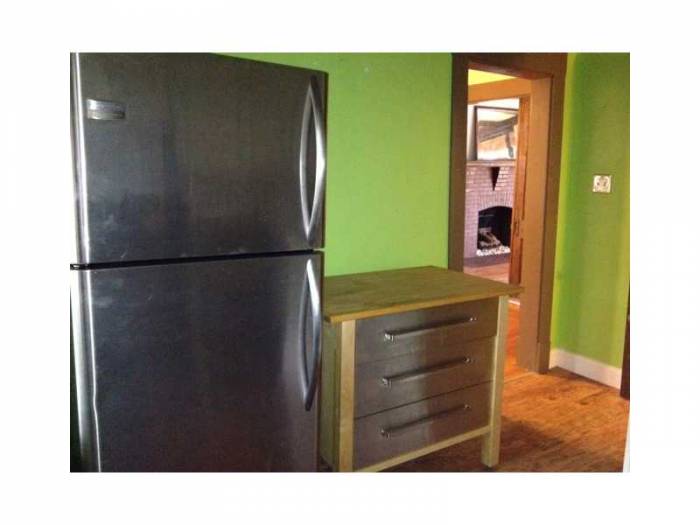The indoor color photograph captures a section of a kitchen area characterized by a few key features. In the left corner, there is a dark slate gray refrigerator with silver handles on the right side, likely a smaller model with the freezer compartment on top and the refrigerator section below. Directly to the right of the refrigerator, positioned centrally in the image, is a chest of drawers with three compartments, each adorned with long, thin rectangular handles. The top of this chest is a flat wooden surface, possibly a butcher's block, suggesting it could serve as additional workspace or storage for kitchen items. Both the refrigerator and the chest of drawers are set against a bright green wall, accented with white trim. To the far right, there is an open doorway leading to another room where a brick fireplace is visible. This fireplace features a mantle adorned with a painting. The floor throughout the scene is hardwood, and the photograph possesses a slightly grainy texture with no text or printed words.